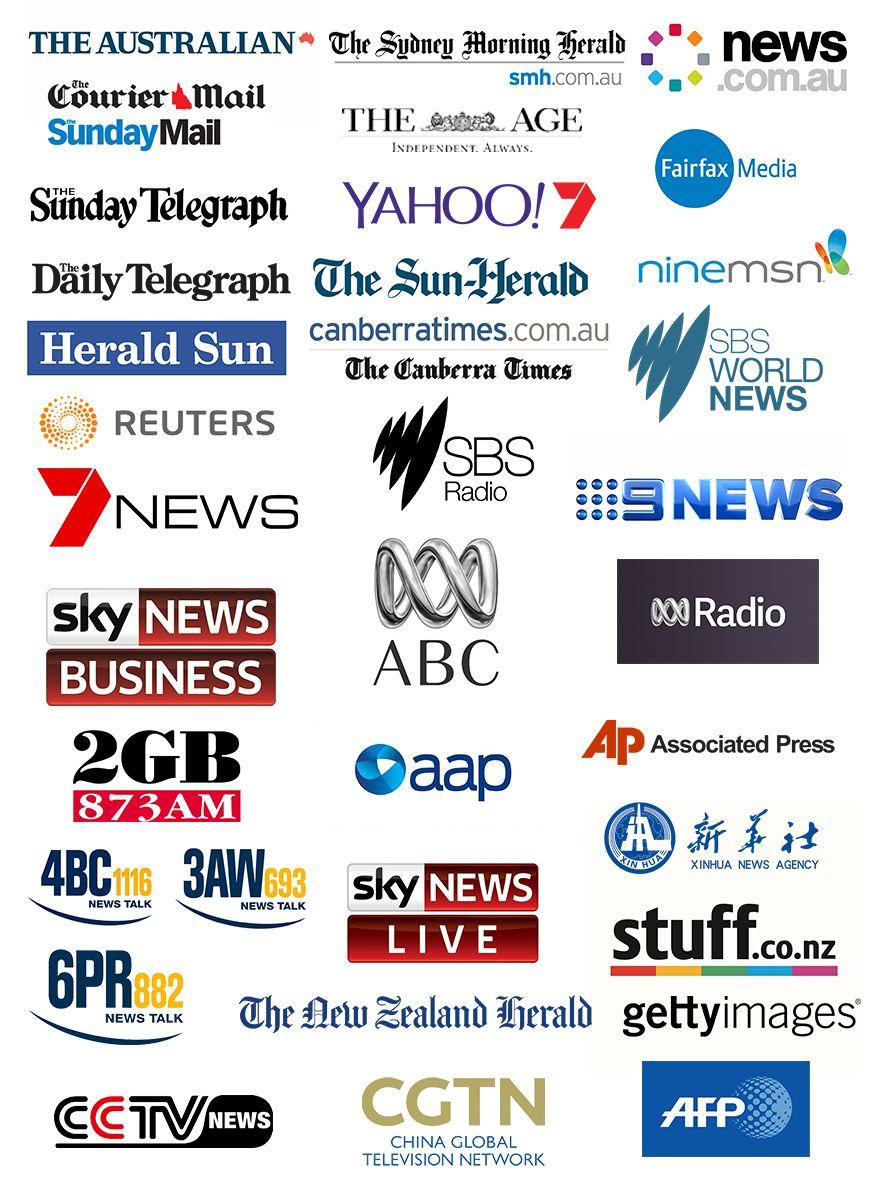This image features an organized display of various media company logos arranged in three columns against a white background. Here is a detailed breakdown of each column top-to-bottom:

**First Column:**
1. The Australian (Blue text)
2. The Courier Mail (Black text)
3. The Sunday Mail (Blue "The Sunday" and Black "Mail")
4. The Sunday Telegraph (Black text)
5. The Daily Telegraph (Black text)
6. The Herald Sun (Blue background, White text)
7. Reuters (Gray text, R-E-U-T-E-R-S)
8. Seven News
9. Sky News Business
10. 2GB 873 AM
11. 4BC 1116 News Talk
12. 3AW 693 News Talk
13. 6PR 882 News Talk
14. CCTV News

**Second Column:**
1. The Sydney Morning Herald (Black text), followed by "smh.com.au"
2. The Age (Black text) with the tagline "Independent Always"
3. Yahoo (Red Ribbon/Seven)
4. The Sun Herald (Blue Text)
5. The Canberra Times
6. SBS Radio
7. ABC
8. AAP
9. Sky News Live
10. The New Zealand Herald
11. CGTN (China Global Television Network)

**Third Column:**
1. news.com.au
2. Fairfax Media
3. Nine Entertainment Co. (possibly indicated as "9Emerson")
4. SBS
5. World Order
6. Nine News
7. Infinite Radio (potentially "Infiniate Radio")
8. AP (Associated Press)
9. XINHUA News Agency
10. Stuff.co.nz
11. Getty Images
12. AFP (Agence France-Presse)

Each logo is clearly labeled, reflecting a diverse range of media outlets spanning newspapers, radio, television, and online news portals from various parts of the world.